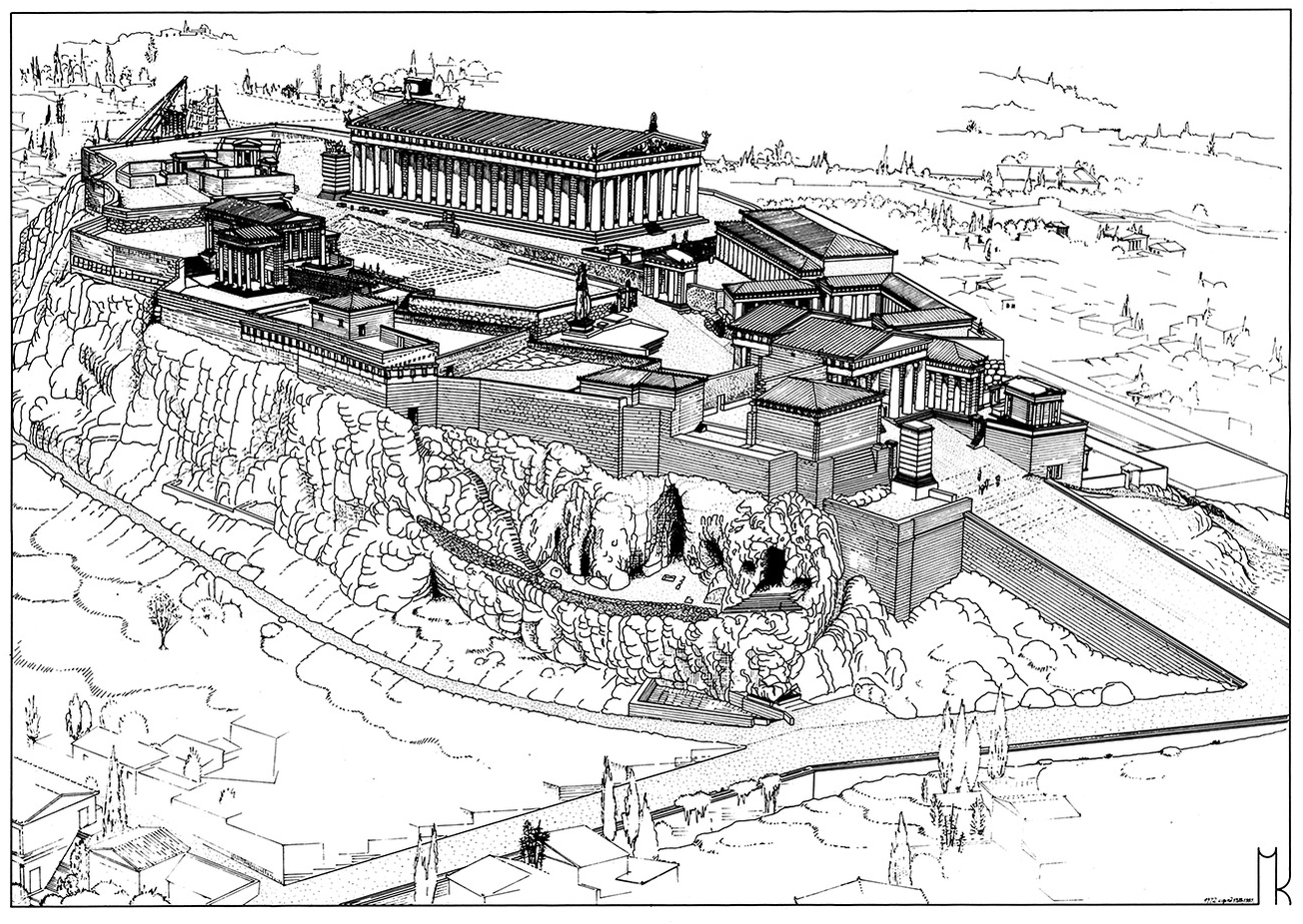The image is a detailed black and white pen and ink sketch depicting a grand architectural complex, possibly an interpretation of the Parthenon and its surrounding structures. Situated on the top or side of a mountain, the drawing features multiple roads and pathways converging in the lower right-hand corner, ascending towards an impressive set of buildings in the upper left. The composition showcases a prominent stairway leading to these grand edifices, which include ornate structures with columns, reminiscent of the Parthenon and perhaps akin to the Jefferson Memorial in their classic design. Scattered smaller buildings and discernible details such as statues and parkways further enrich the scene, lending a sense of historical and civic significance to the area. The focus on architectural details, including partial construction, enhances the impression of a powerful, governing city set against a stark, minimalistic background, emphasizing the monumental nature of the complex.